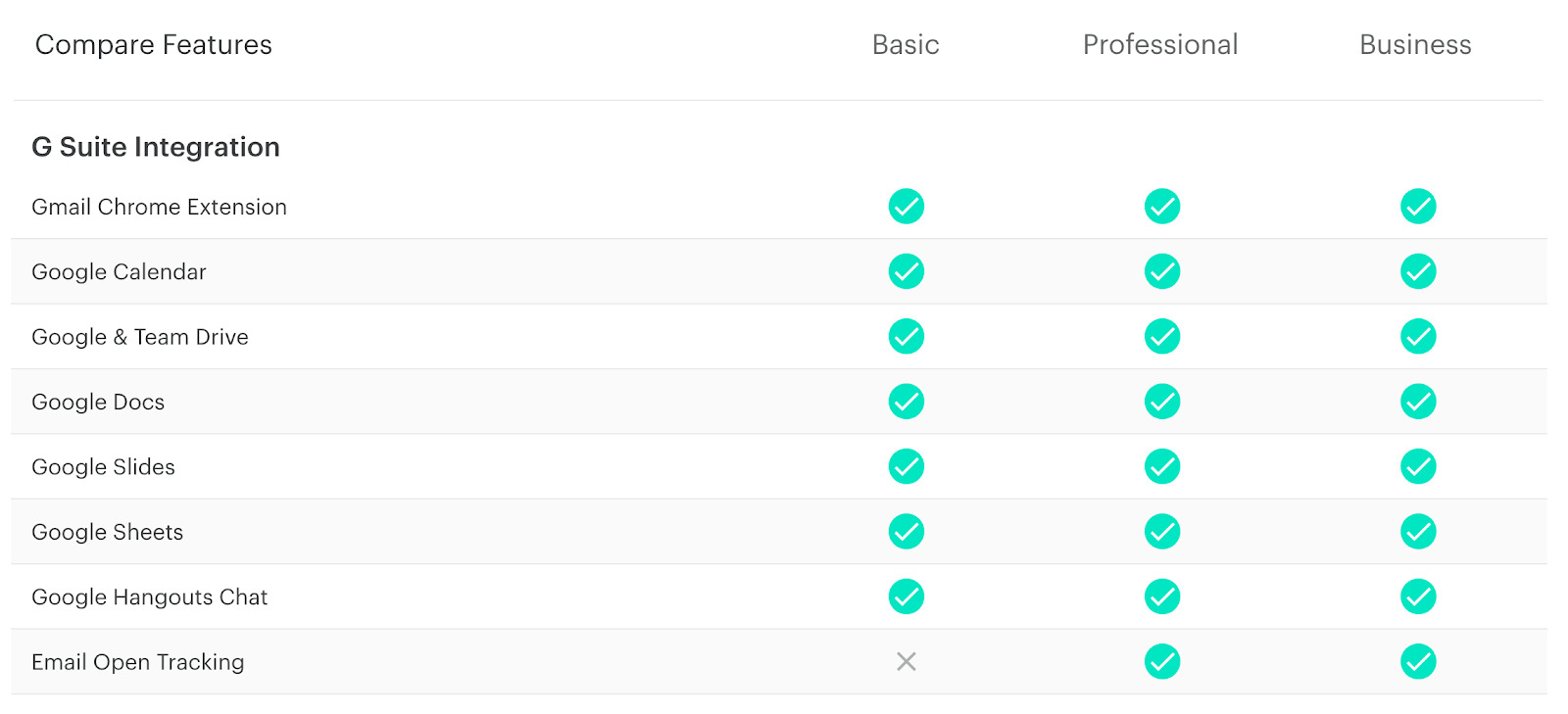The image depicts a web page designed for comparing features of different service plans, similar to how one might evaluate streaming service options. At the top left corner, it prominently displays the heading "Compare Features". The comparison table is divided into three columns labeled "Basic", "Professional", and "Business", from left to right.

Beneath the main headings, a light gray line separates the title from the detailed feature list. The first feature listed is "G Suite Integration", highlighted in bold. Following this, a series of G Suite-compatible services are outlined in smaller, dark gray text. These services include:

- Gmail Chrome extension
- Google Calendar
- Google Team and Drive
- Google Docs
- Google Slides
- Google Sheets
- Google Hangout Chat
- Email open tracking

Each feature is checked for availability using a green, solid bubble with a white check mark, indicating that the feature is included in the respective plan. Notably, the "Basic" plan does not include "Email open tracking", which is marked with a gray X instead.

To enhance readability, the background of the list alternates between white and light gray for each line, making it easier to distinguish individual features.